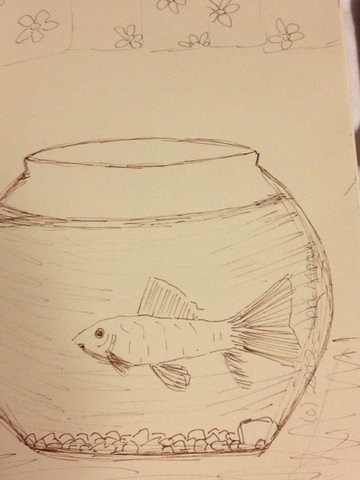This image features a detailed pencil drawing on yellowish paper, depicting a goldfish inside a classic circular fishbowl, commonly found in pet stores. The goldfish, meticulously drawn with a small mouth, a visible eye, and distinct gills, holds its body perfectly straight horizontally, showcasing three pronounced fins including a dorsal fin. Its fins and whiskery gill details add realism to the scene. At the bottom of the fishbowl, there are scattered pebbles or decorative rocks, with shaded water making the bowl appear slightly darker than the glass itself. The fishbowl rests on a surface suggested by lines and shading that indicate a tabletop. Above the fishbowl, near the top edge of the paper, is a border adorned with six abstract daisy blossoms, each flower featuring five petals and a central circle, possibly representing a curtain or decorative element. The entire piece showcases skilled hand-drawn lines and shading techniques.